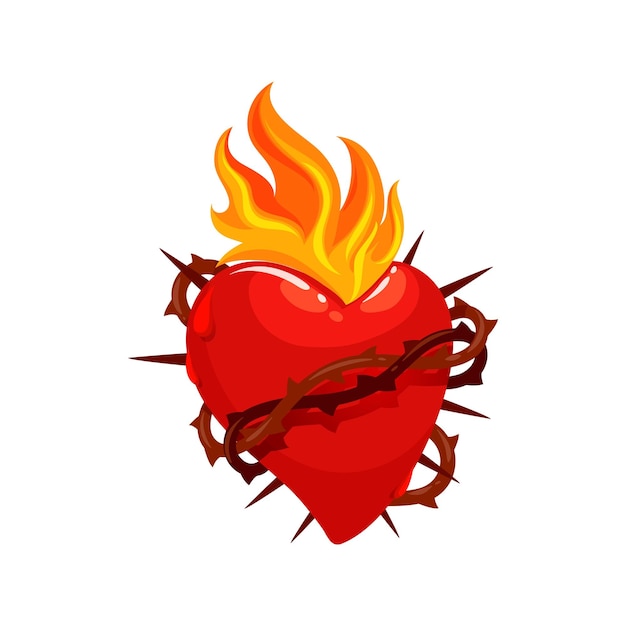The image depicts a stylized, cartoonish red heart that transitions from a lighter hue at the top to a darker shade at the bottom. The heart is adorned with intertwined barbed wire—one strand is brown, while the other is black—that wraps around its middle, both at the front and the back. Some portions of these wires feature spikes or barbs, which add to its rugged appearance. At the top of the heart, there is a flame with a yellow base that shifts to an orange tip, adding a fiery dimension to the image. Additionally, numerous sharp spikes protrude from the back of the heart, with specific arrangement: four on the left (two at the top and two at the bottom) and five on the right (two at the top and three at the bottom). Overall, the heart evokes the imagery of a flaming, barbed-wire-wrapped emblem, possibly reminiscent of a tattoo design.